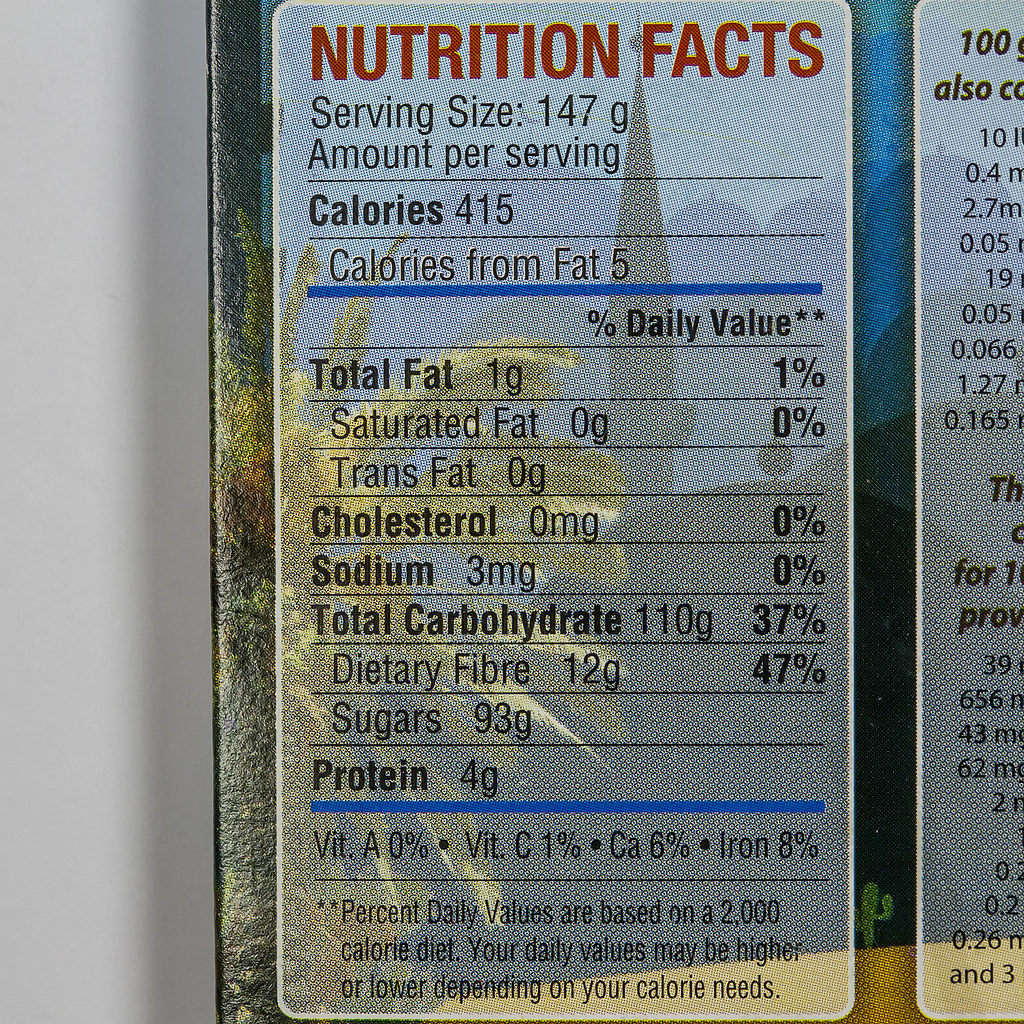This detailed close-up image prominently features the Nutrition Facts label found on the back of a food package. The Nutrition Facts heading is bold and in red, drawing immediate attention. Below this heading, the detailed nutritional information is listed. The serving size is specified as 147 grams, with a total caloric content of 415 calories, including 5 calories from fat. 

On the right side of the image, part of another label is visible, though not entirely readable, indicating that the packaging might contain additional information or branding. The left edge of the package marks the boundary of the image, showcasing a vertical white strip spanning from the top to the bottom of the frame, occupying approximately 20% of the image. This strip, alongside the Nutrition Facts label, offers a comprehensive view into the nutritional profile of the product while providing a glimpse into the design and layout of the packaging.